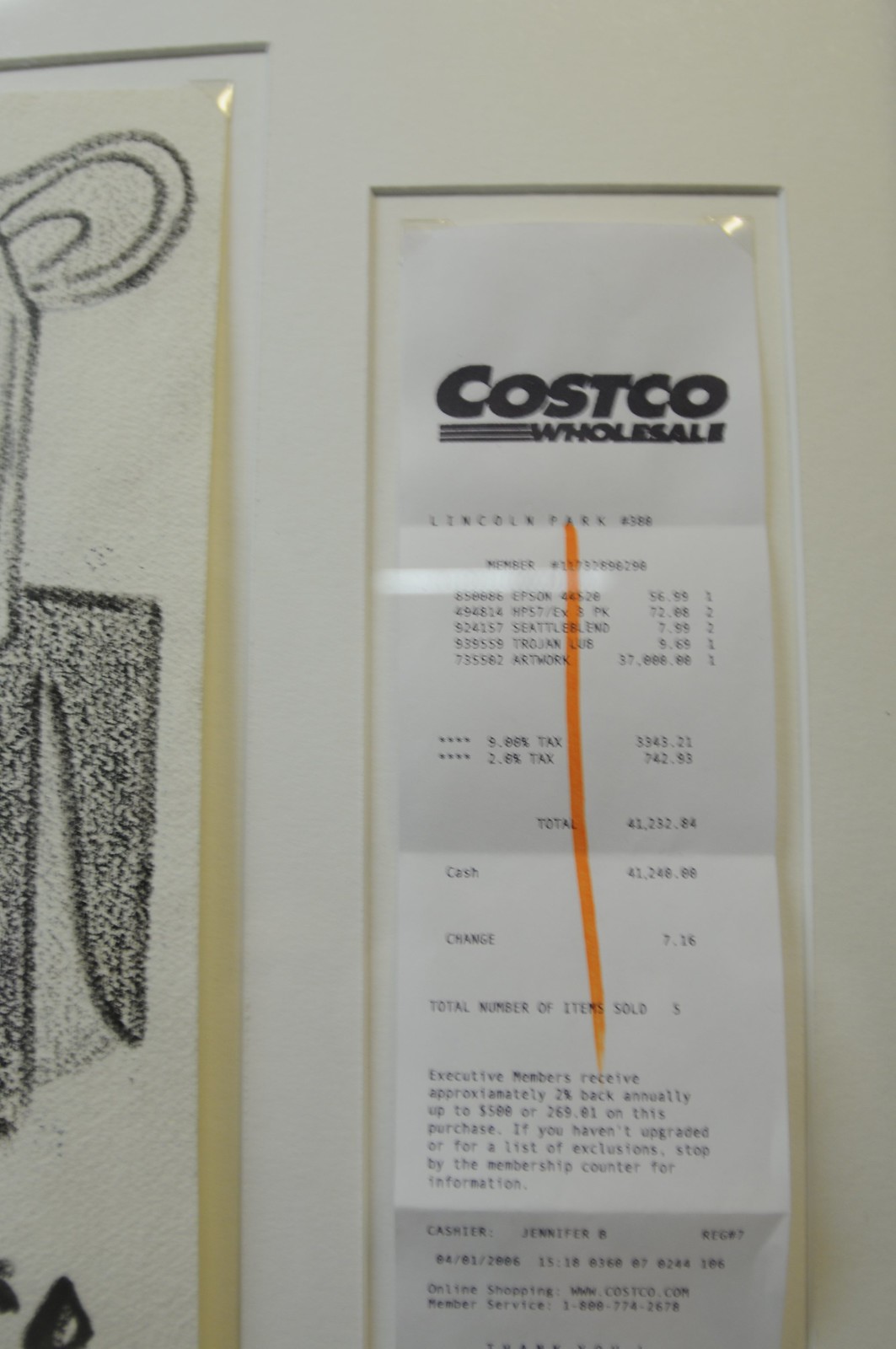This image depicts a scene with two white picture frames mounted on a wall. In the larger frame, positioned on the left side but only partially visible, there's a portion of what appears to be a pencil-drawn artwork, potentially a child’s simplistic stick figure drawing. The main focus is on the right-side frame, which is vertically oriented, rectangular in shape with a greater height compared to its width. Within this frame, a folded Costco wholesale receipt is displayed, prominently marked by a vertical orange slash, indicative of the store’s verification process by a checker. The receipt details a substantial purchase totaling $41,240, although the specific items are not easily discernible. The frames both feature a shiny, reflective surface that complements their clean, white appearance.